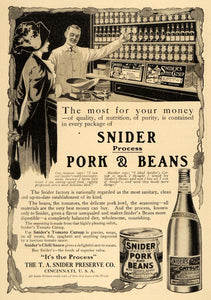The image appears to be a scanned advertisement from an old magazine or an advertising circuit, featuring slightly browned paper and an ink illustration. At the top, the prominent heading reads, "The most for your money," followed by smaller, mostly illegible text. Below, in large, bold black text, it announces "Snyder (SNIDR) presents pork and beans," using the '&' symbol for 'and.' Additional smaller text surrounds the main text, including a tagline at the bottom, "Snyder pork and beans," displaying an illustrated can and a tall glass bottle with an unreadable sticker.

The illustration depicts a scene where an older shopkeeper, dressed in white, points towards shelves filled with Snyder pork and beans and other food items. He appears to be presenting these goods to a wealthy-looking woman, who is wearing a grand black dress and a large black hat adorned with white flowers. At the bottom, a quote reads, "It's the process," attributed to the T.A. Snyder Preserve Company, Cincinnati, USA.